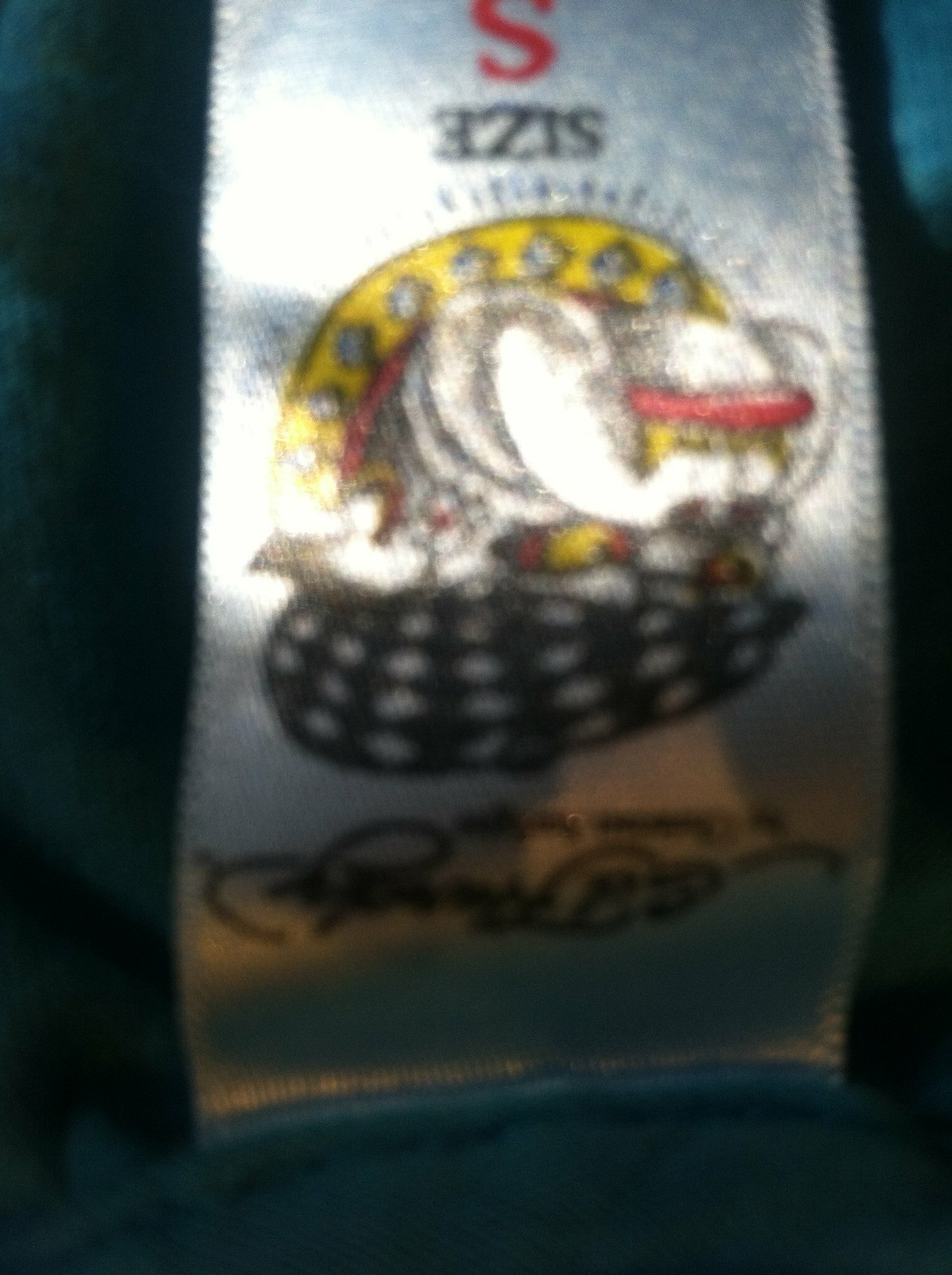This is a blurry, close-up photograph of the inside label of a garment, located at the neck. The label appears white against the dark blue fabric of the clothing, accentuated by white stitching around it. The label is notably shiny and silky, and it's positioned upside down in the image. The main readable text on the label is "size small," with "size" written in black and "S" in red. The label also features a detailed but unclear illustration. Despite the blurriness, the illustration seems to depict a fierce-looking bulldog with white jowls, a red tongue, and yellow, spiked teeth. The bulldog has yellow eyes and is adorned with a yellow spiked collar. It is also wearing a small hat, black and white with a checkered pattern and a brim with a dot on top. The drawing is quite intricate and colorful, combining black, yellow, red, and white. Despite the overall blurriness, these distinct elements are partially discernible.